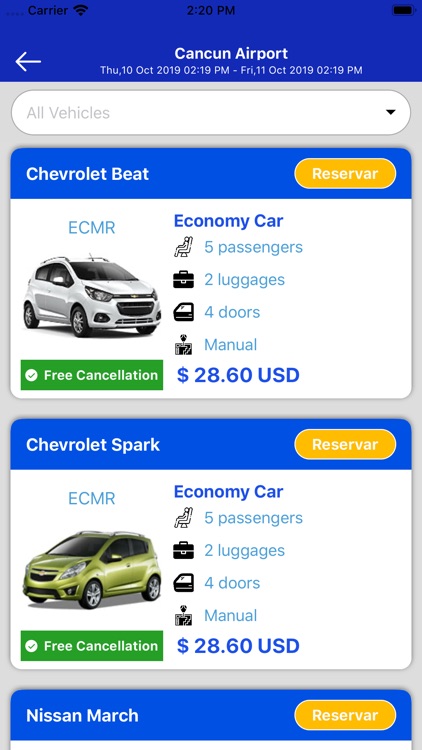A detailed screenshot captures a mobile phone display at Cancun Airport on Thursday, October 10, 2019, at 2:19 p.m. The phone status shows a full battery and a strong Wi-Fi connection on the carrier "P.M." The background of the phone screen is black with white text displaying the date and time.

The screenshot is taken from a rental car reservation webpage, detailing available vehicle options at the Cancun Airport from Thursday, October 10, 2019, to Friday, October 11, 2019, at 2:19 p.m.

1. **First vehicle option:**
   - **Car Model:** Chevrolet Beat ECM
   - **Type:** Economy Car
   - **Capacity:** 5 passengers
   - **Luggage:** 2 pieces
   - **Doors:** 4
   - **Transmission:** Manual
   - **Special Feature:** Free Cancellation (indicated by a green checkmark)
   - **Price:** $28.60 USD

2. **Second vehicle option:**
   - **Car Model:** Chevrolet Spark
   - **Type:** Economy Car
   - **Capacity:** 5 passengers
   - **Luggage:** 2 pieces
   - **Doors:** 4
   - **Transmission:** Manual
   - **Special Feature:** Free Cancellation
   - **Price:** $28.60 USD
   - **Image:** Picture of a silver car

3. **Third vehicle option:**
   - **Car Model:** Kia Hatchback
   - **Color:** Green

4. **Fourth vehicle option:**
   - **Car Model:** Nissan March
   - **Special Feature:** Free Cancellation (indicated by white lettering with a yellow highlight)

The webpage shows no other options or additional information. The user expresses a sentiment, noting the affordable prices of rental cars in Cancun compared to those in the United States.